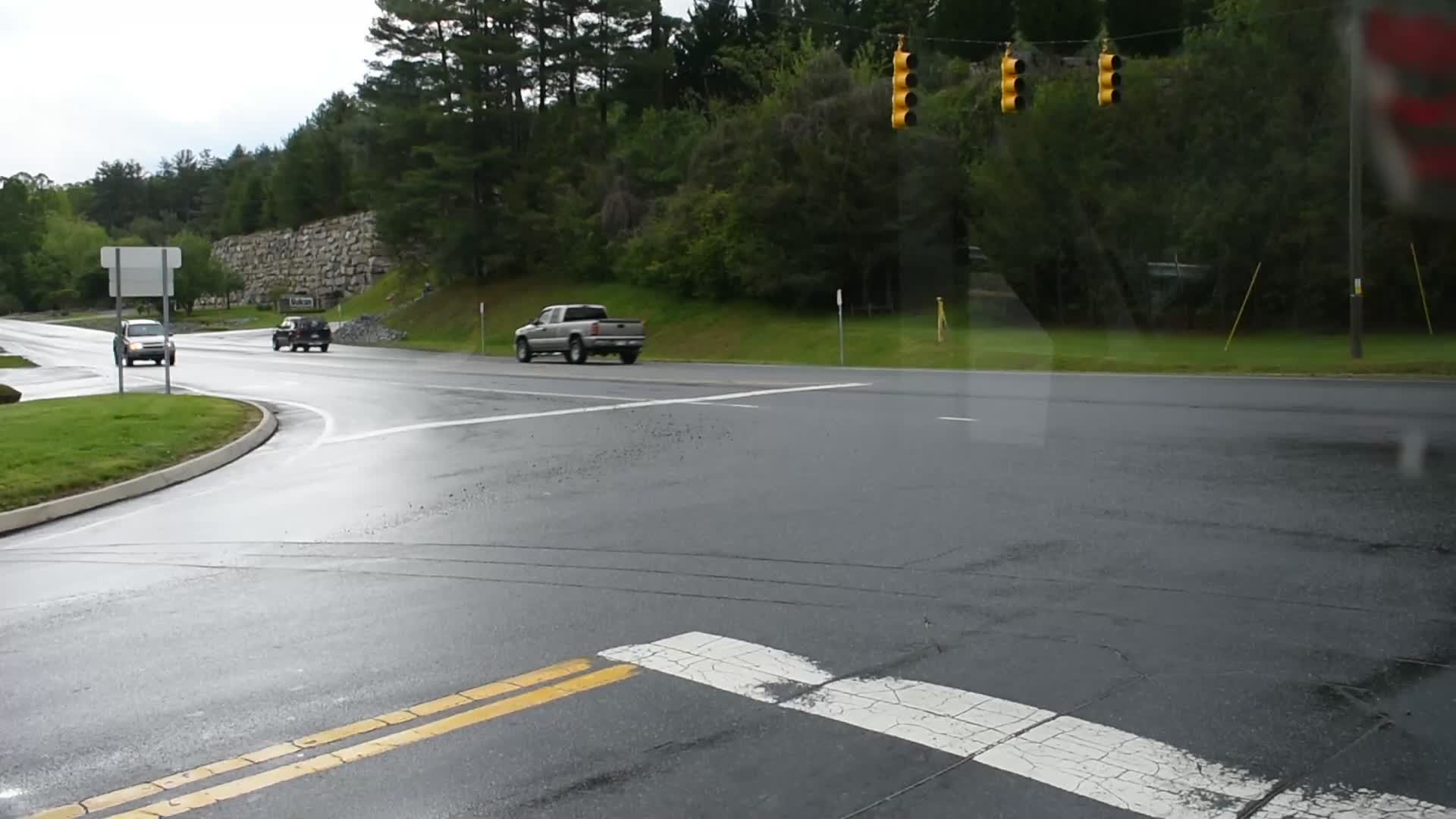The photograph captures a busy intersection where one road, emerging from the lower left-hand side, meets another road at a T-junction. Overhead, streetlights are suspended at the center of the intersection, providing illumination for the converging roads. To the left, a road branches off, leading towards a verdant landscape filled with grass and trees. In the background, a stone wall is visible towards the upper left-hand corner, adding a rustic touch to the scene. Additionally, a street sign is partially seen from the back. The intersection is occupied by three vehicles: a silver pickup truck, a Subaru Outback, and another car resembling a Honda, all converging towards the junction. The overall setting presents a slice of suburban life, framed by natural greenery and human-built infrastructure.